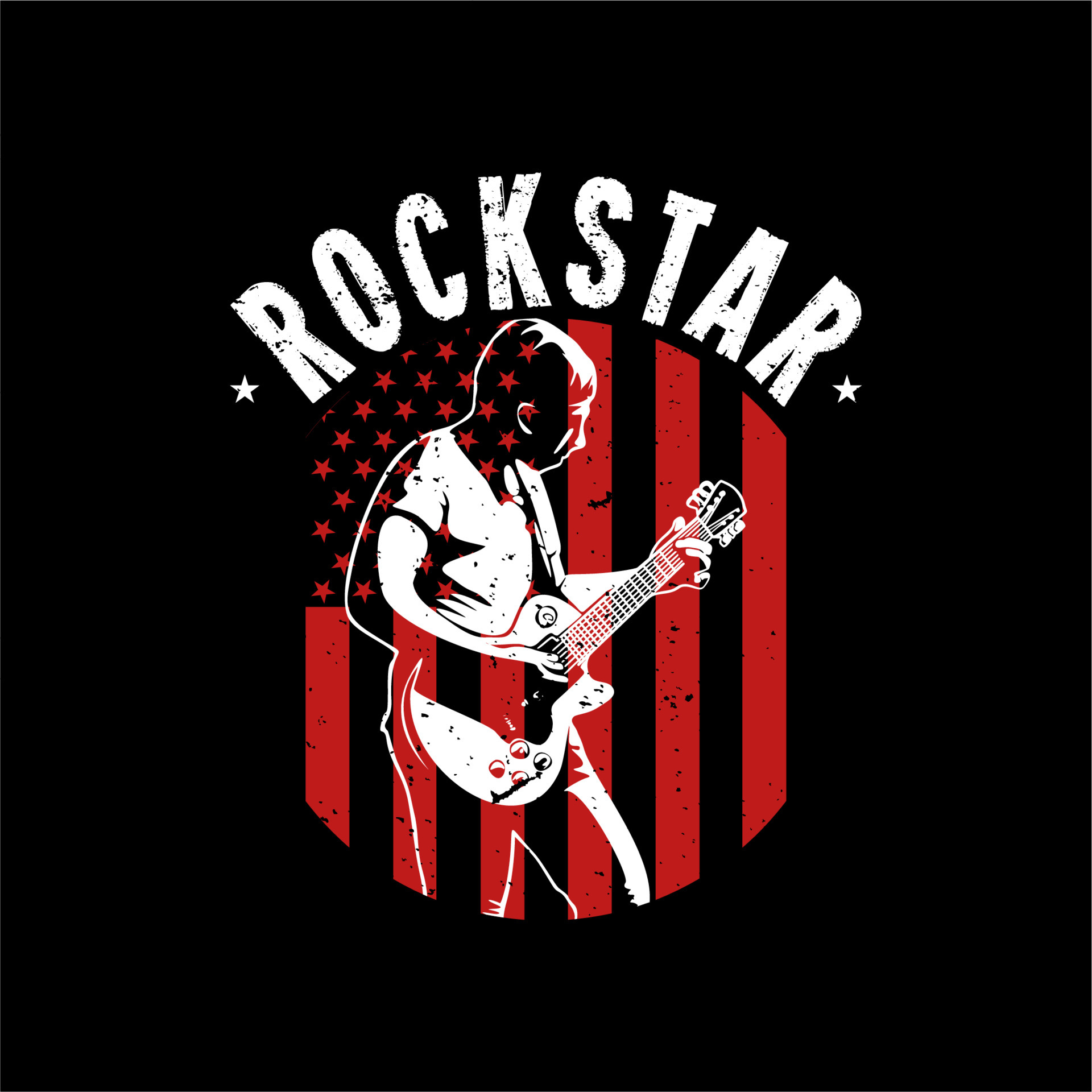The image, resembling a large poster, has a solid black background and is centered with bold, white text that arcs upwards, spelling "Rockstar." Flanking the text on either side are small white stars. Below the lettering, centrally positioned, is an oval or egg-shaped depiction of the American flag rotated 90 degrees, so its red, vertical stripes and red stars on the upper left are visible. Superimposed or interwoven with this flag is a stylized, white-outlined, digitally drawn man strumming an acoustic guitar. His short hair and precise details are indistinct due to the monochromatic white rendering. The entire composition emphasizes the iconic "Rockstar" theme, focusing on a solitary musician and an abstracted version of the American flag, emphasizing a stark color scheme of red, white, and black.